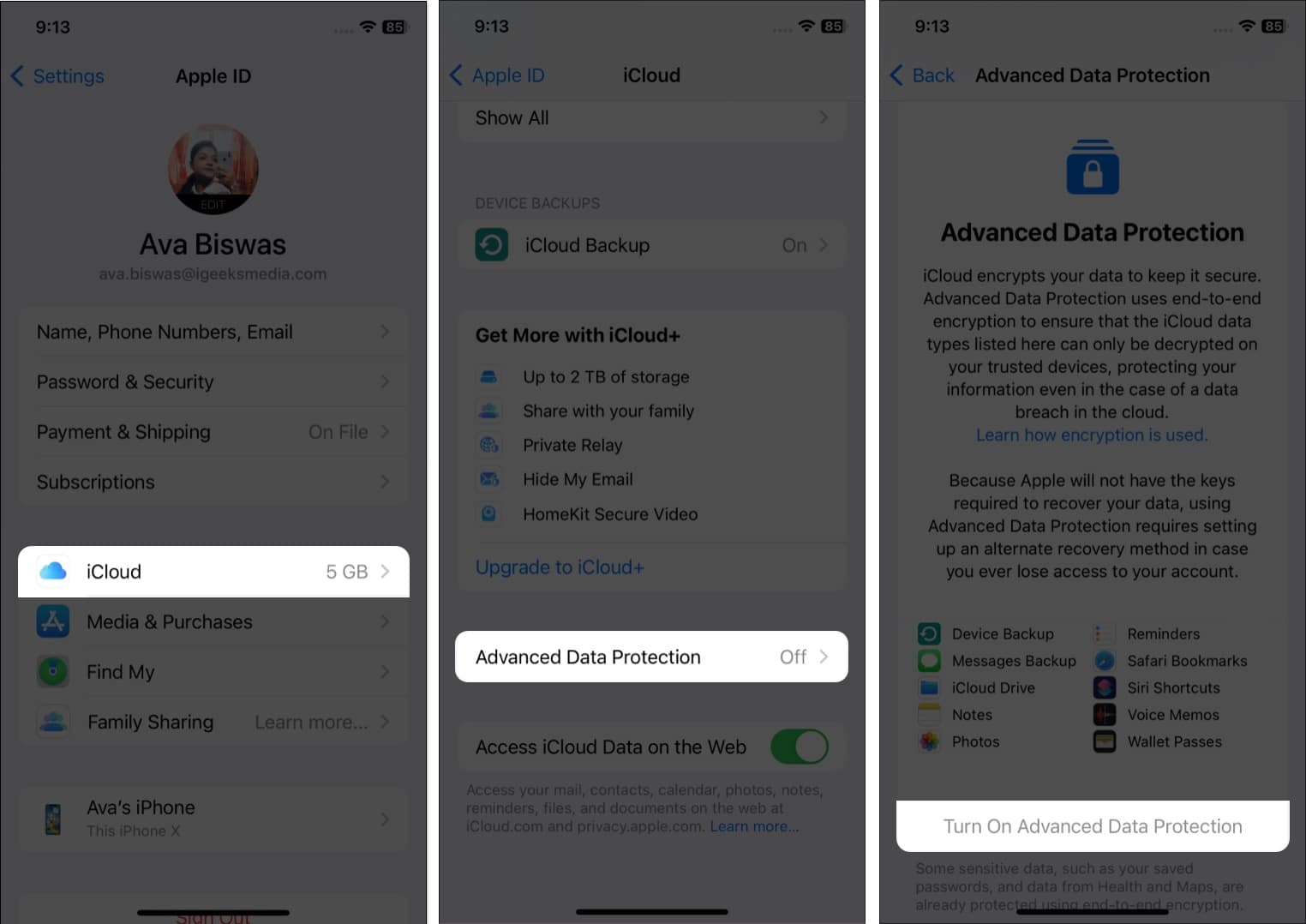This is a set of three sequential images displayed in a horizontal format, each portraying a screenshot of an iPhone's settings interface. 

1. **First Screenshot:** The image captures the Apple ID settings screen on an iPhone. Most of the screen is grayed out with the exception of the "iCloud 5GB" section, which is highlighted, drawing attention to that specific part. The top of the screen reads "913 Settings," followed by the user’s Apple ID details: "Ava Biswas, ava.biswas@igeekmedia.com." Various options are listed, such as "phone numbers," "email," "password and security," "payment and shipping," "subscriptions," and "media and purchases." There's further mention of "Find My," "Family Sharing," and "Learn More." The device name "Ava's iPhone" along with the model, "this iPhone X," is also visible.

2. **Second Screenshot:** This screenshot dives deeper into the iCloud settings. Similar to the first image, the background is grayed out, emphasizing the section "Advanced Data Protection" which has been highlighted. The screen includes headings like "Apple ID" and "iCloud," with an option to "Show All." The "iCloud Backup" feature is turned on, indicated by the slider button. Promotional text about iCloud+ offers up to 2TB of storage, family sharing, Private Relay, "Hide My Email," and HomeKit Secure Video is visible. The section about "Advanced Data Protection Off" is highlighted, suggesting the user can upgrade to iCloud+ for extra features. 

3. **Third Screenshot:** This final image elaborates on "Advanced Data Protection." It explains that iCloud uses end-to-end encryption to keep data secure, implying that only trusted devices can decrypt certain types of iCloud data. The section clarifies that more secure data handling prevents unauthorized access even in a potential cloud data breach. The user is informed about the necessity of setting up an alternate recovery method due to Apple not retaining recovery keys. Listed items include "Device backup," "Messages backup," "iCloud Drive," "Notes," "Photos," "Reminders," "Safari bookmarks," "Siri shortcuts," "Voice memos," and "Wallet passes." A specific section on learning how encryption works is highlighted, emphasizing its importance.

Each image progressively focuses on enabling and explaining the Advanced Data Protection feature within the iPhone’s iCloud settings.